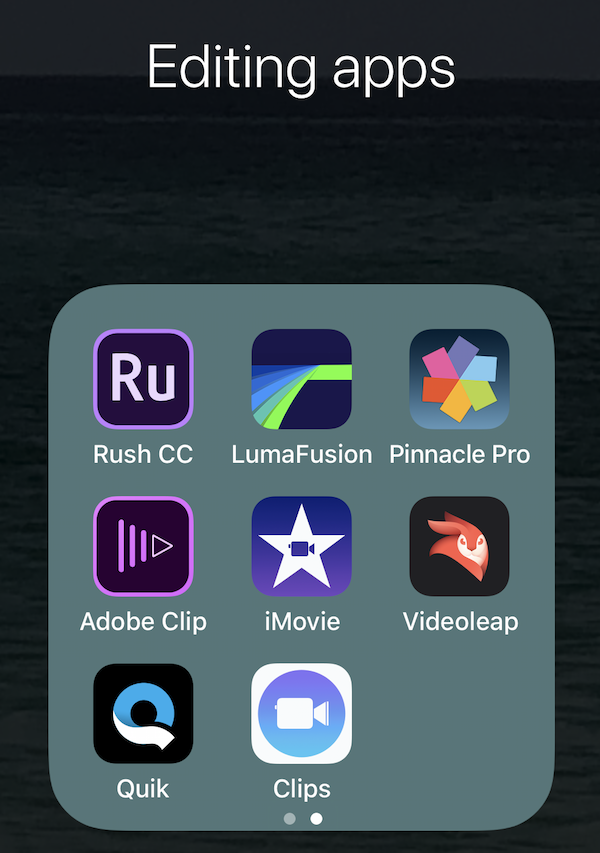The image features a screenshot of a phone screen showcasing a personalized folder labeled "Editing Apps." The folder has a gray background with rounded edges and contains a 3x3 grid displaying eight app icons. From right to left and top to bottom, the apps included are Rust CC, Luma Fusion, Pinnacle Pro, Adobe Clip, iMovie, Video Leap, Quik, and Clips. At the bottom of the folder are two small dots, indicating there are additional pages or sections within this folder. The screenshot captures the action of someone selecting or highlighting the folder to showcase the specified editing apps.